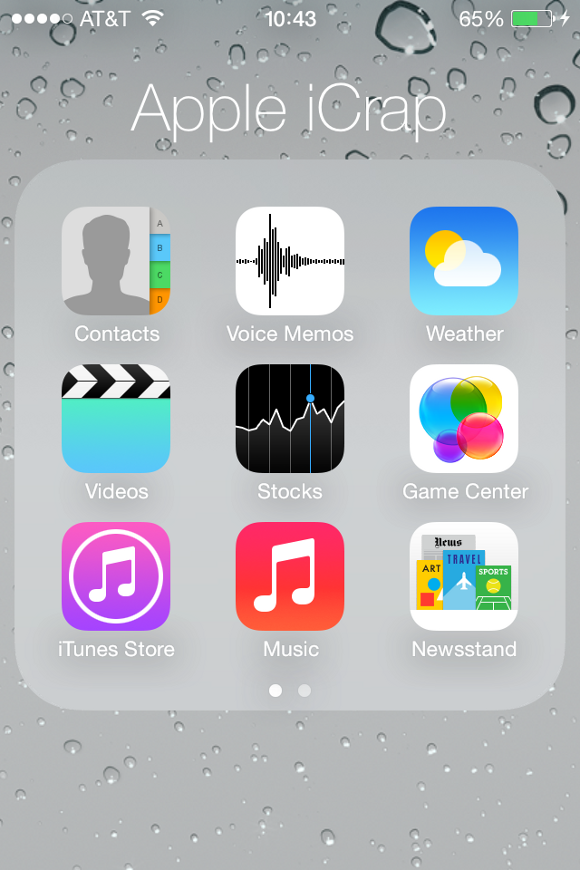The image is a screenshot from an Apple device displaying a folder titled "Apple iCrap." The folder contains nine app icons:
1. **Contacts** - Illustrated by a silhouette of a person with the letters ABCD descending down the right.
2. **Voice Memos** - Depicted with an image of a microphone.
3. **Weather** - Shows a blue sky with a white cloud partially covering a yellow sun.
4. **Videos** - Represented by a filmmaker's clapboard.
5. **Stocks** - Displays a bar graph indicating stock performance.
6. **Game Center** - Illustrated with colorful bubbles in pink, purple, yellow, and blue.
7. **iTunes Store** - Shows music notes inside a white circle on a purple background.
8. **Music** - Depicted by music notes on a red background.
9. **Newsstand** - Displays images of various magazines.

At the top, the status bar indicates a few device details: it is 10:43, the device is connected to Wi-Fi, has AT&T as the service provider, and has a 65% battery charge.